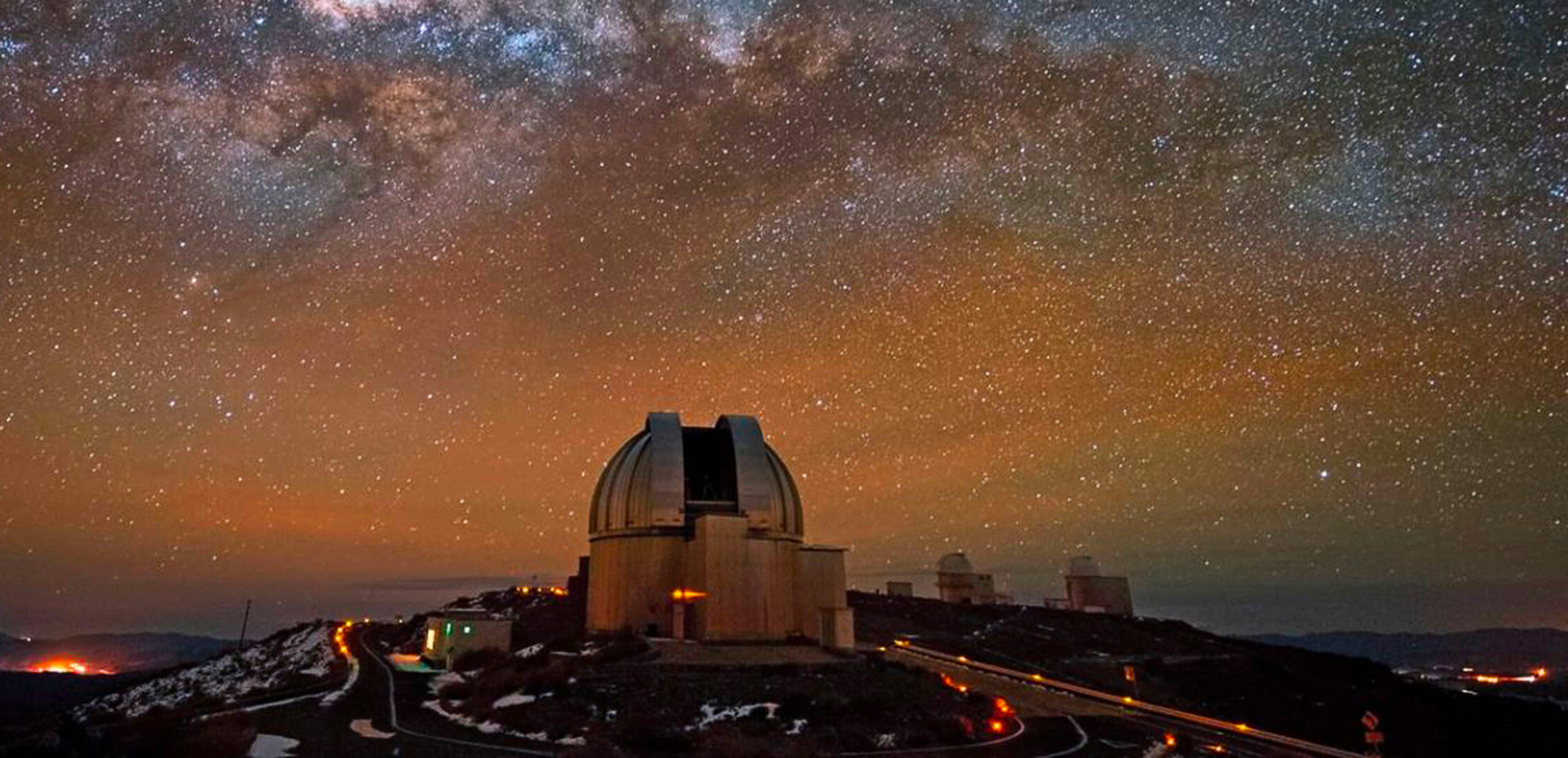In this photo, taken at nighttime, a grand observatory dominates the scene, perched atop a dark, slightly domed hill. The observatory, with its large white stone base and prominent dome-shaped top, is illuminated against a mesmerizing night sky. The sky itself is an intricate tapestry of colors—brownish-red, orange, and blue—accompanied by a multitude of glittering stars that create a smoky, almost ethereal ambiance. Surrounding this central structure are several smaller buildings, including a small stone square building to the left. A lit highway winds its way up the hill, marked by tiny orange lights that guide the way. In the background, a few additional orange lights punctuate the landscape, completing this breathtaking nocturnal scene.